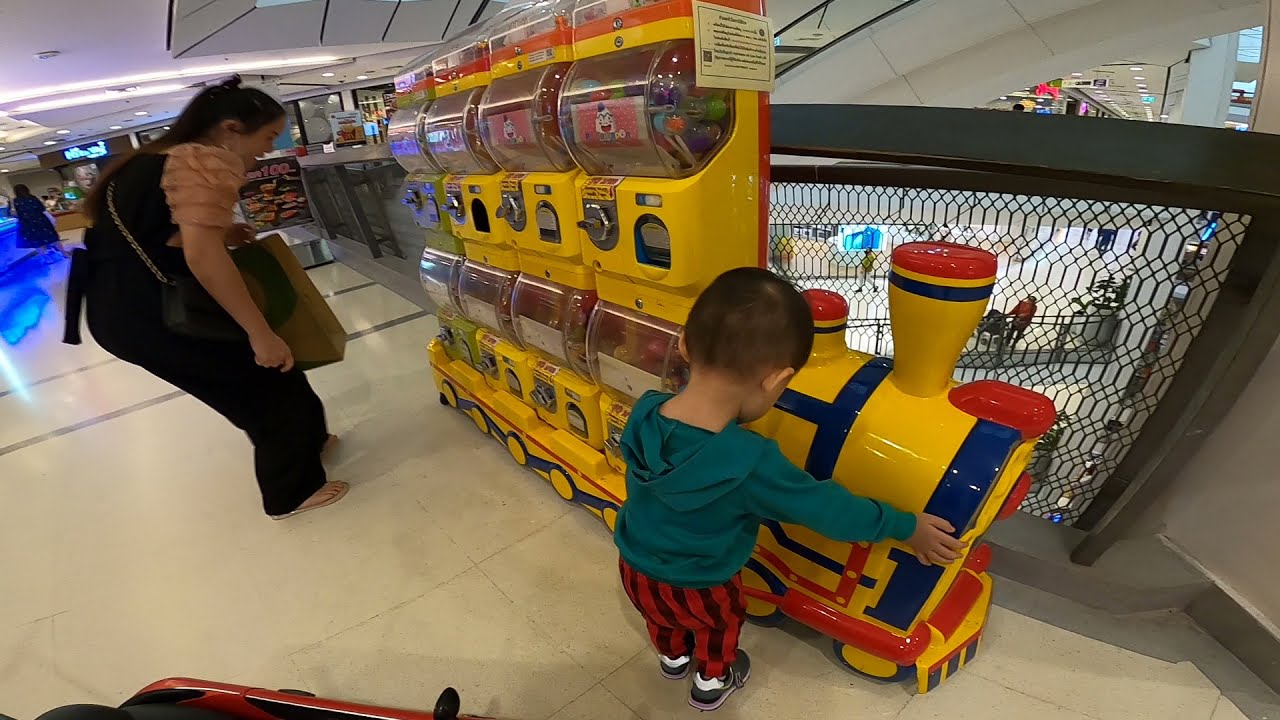The image captures the interior of a multi-storied mall, focusing on a young child who appears to be a boy, dressed in a green hoodie paired with red striped pants and black tennis shoes. He is engaged with a unique vending machine designed to resemble a yellow train with blue and red accents, containing a total of eight sections for dispensing toys or candies upon inserting coins. The boy is looking down, fascinated by the train-shaped machine, while a woman stands to his left. She is dressed in a pink and black blouse, black pants, and rose gold-colored sandals, and seems to be considering which option to choose from the vending machine. A railing in the background indicates the elevated floor, with a white and gray color scheme dominating the mall's interior.